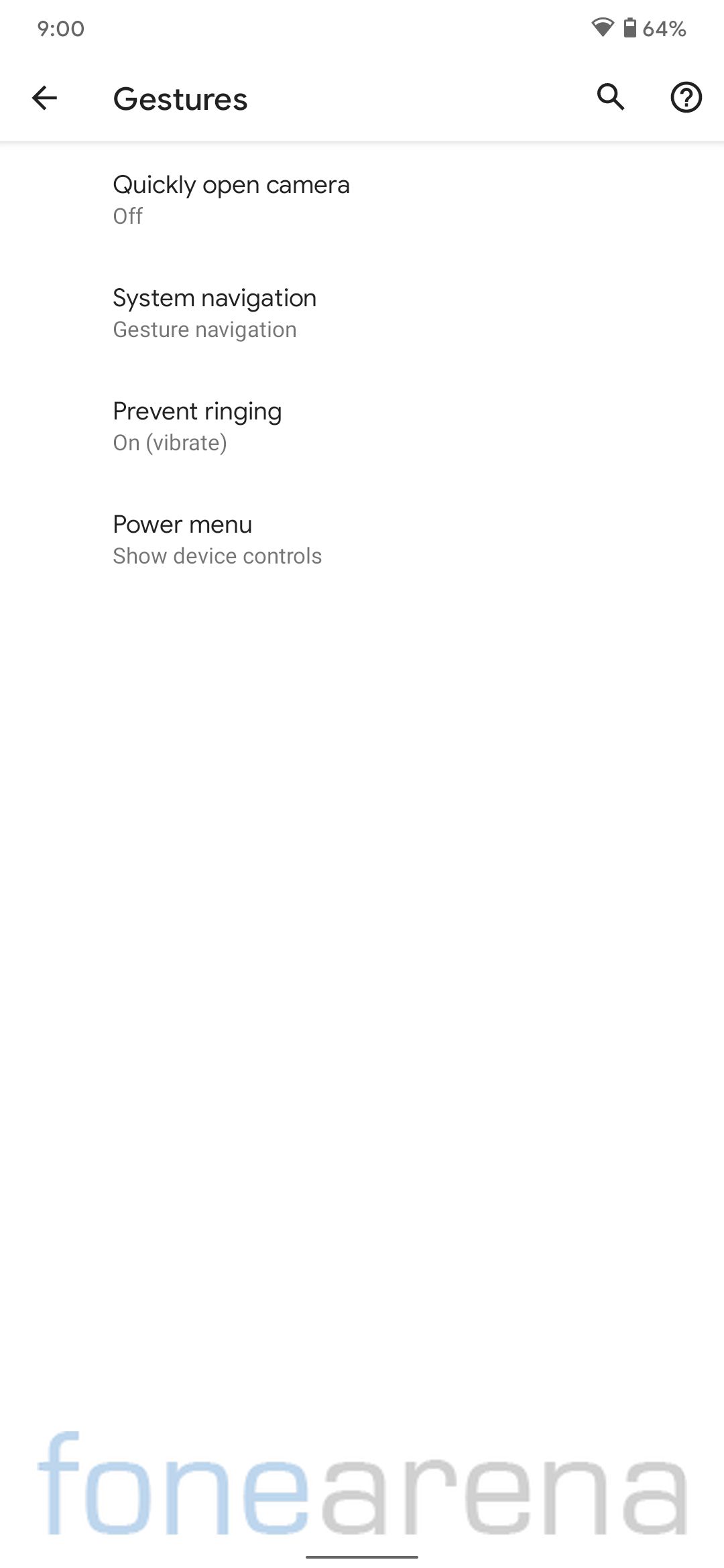This image is a vertically oriented screenshot taken on a mobile device with a white background. The image appears slightly stretched and has low resolution, causing some text to look grainy. Zooming in slightly improves the resolution but it remains imperfect. 

In the top left-hand corner, the time displayed is 9:00. In the top right-hand corner, the battery level is shown as 64% charged. Below the top bar, on the left-hand side, there is a black back arrow pointing to the left next to the word "Gestures" in black text. On the right-hand side of this section, there is a black search icon and a black circle with a black border, inside which there is a black question mark.

Beneath this, a thin vertical line spans from the left-hand side to the right-hand side, separating it from the menu options below. The menu options include:

- "Quickly open camera" which is set to off.
- "System navigation" set to gesture navigation.
- "Prevent ringing" set to on, with further specification in parentheses (vibrate).
- "Power menu" set to show device controls.

At the very bottom of the image, there is a large text. In blue, it says "FONE" and in gray, it says "ARENA." The first "A" in "ARENA" is underlined in black.